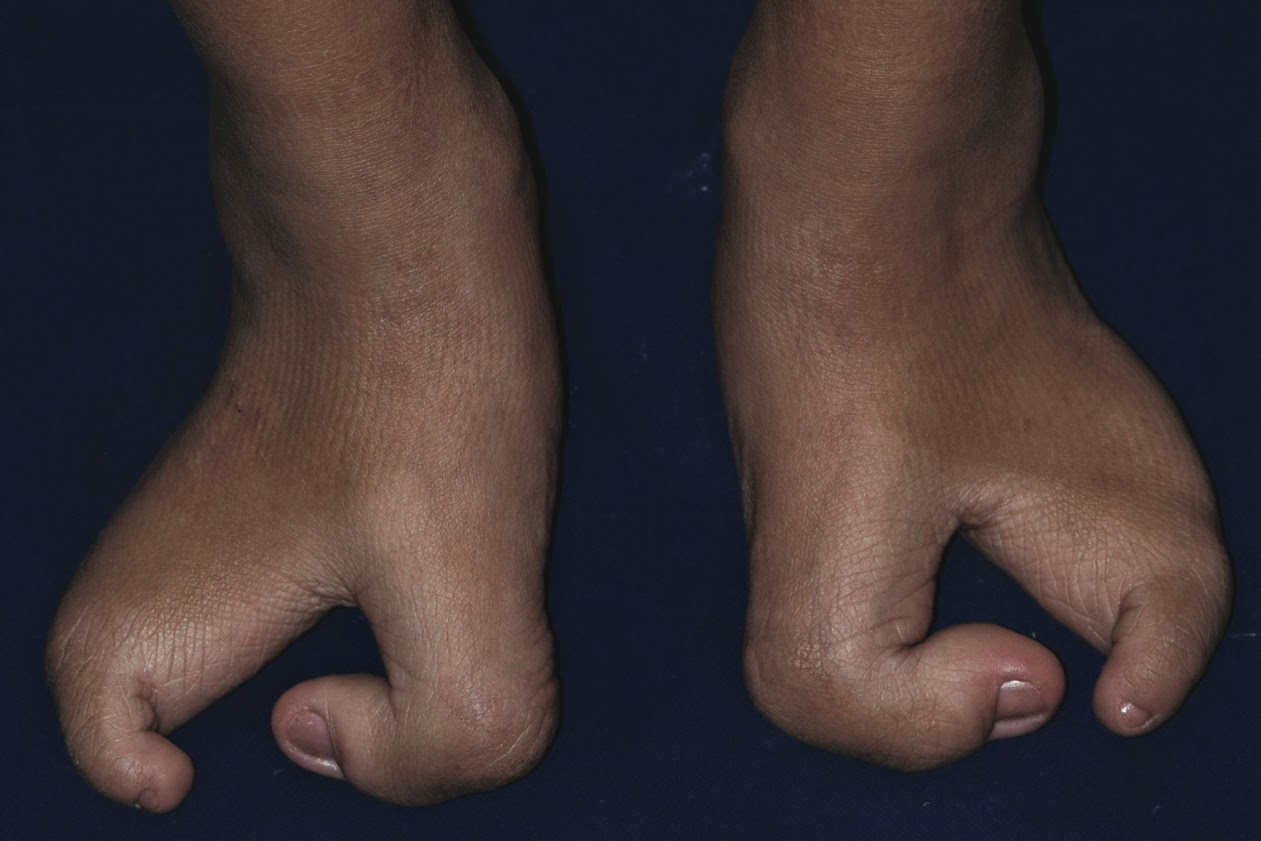This rectangular photograph features a pair of deformed feet against a dark, possibly carpeted background. The feet, centrally positioned in the image, display an unusual deformity—they each have only two toes, a large toe and a small one. The toes curve towards each other, forming a V-shaped space in between. The skin tone is medium brown, and the feet appear somewhat swollen, especially around the ankle area, which is also visible in the photograph. The background is a dark blue surface with small specks, possibly dirt or threads, scattered across it, adding to the sense of a lived-in, somewhat untidy environment.